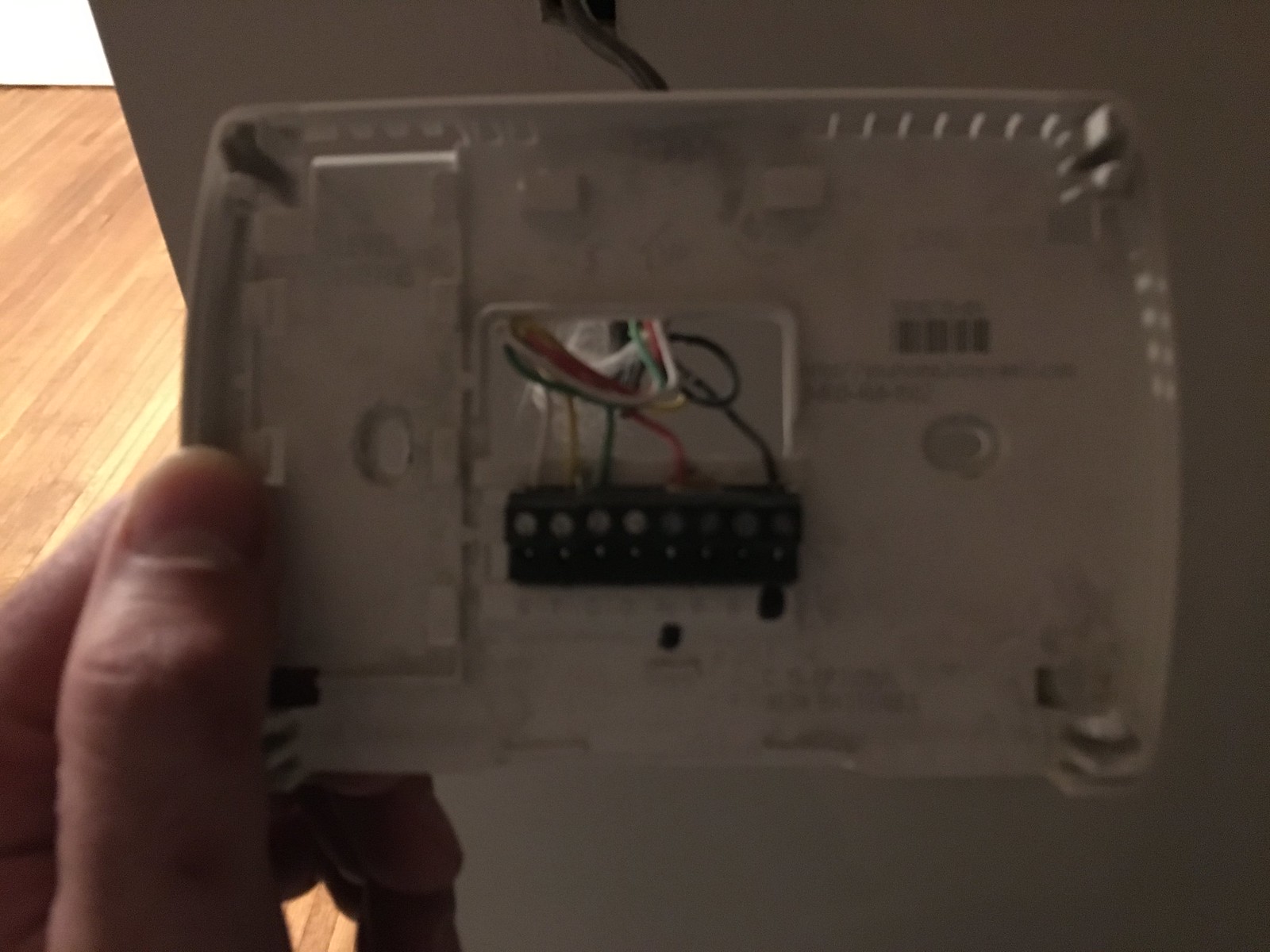A dismantled rectangular device is prominently displayed in the image, revealing its inner components. The device appears to be deliberately unscrewed by someone, allowing a clear view of its interior electronics. Inside, a smaller black rectangular piece is visible, featuring eight circular connectors arranged in a horizontal row. A series of colored wires—red, yellow, white, green, and black—are intricately connected to this black component, indicating a complex internal circuitry. These wires trace back into a small rectangular opening in the white wall behind the device, suggesting a built-in installation. The device is held by a person's left hand, with their thumb and fingers wrapped around the left side, giving a sense of scale and involvement. In the background, to the far left, a light brown wooden floor is partially visible, adding context to the scene. While the exact nature of the device remains unidentified due to the absence of readable text or labels, it closely resembles the back of a thermostat or a similar electronic apparatus.